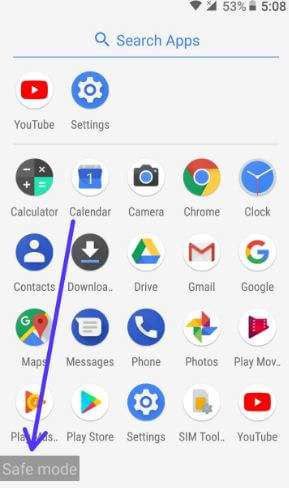**Screenshot Descriptive Caption:**

The screenshot showcases a mobile device with a gray background and predominantly gray font. At the top of the image, there is a Wi-Fi symbol and a signal strength indicator with an 'X' next to it, signifying no signal. The battery level is displayed at 53%, and the time is 5:08.

Below this, in blue text, "Search apps" is displayed alongside a magnifying glass icon, with a blue underline. 

Following this section are various app icons, each with their respective app names in gray font:

1. **YouTube**: Red and white play button logo.
2. **Settings**: Blue and white cogwheel.
3. **Calculator**: Gray, green, and white icon.
4. **Calendar**: Blue and white calendar page icon.
5. **Camera**: Blue and gray camera icon.
6. **Chrome**: Red, green, gold, and blue circular icon.
7. **Clock**: White and blue clock icon.
8. **Contacts**: Blue and white person icon.
9. **Downloads**: White arrow on a blue line within a gray circle.
10. **Google Drive**: Green, gold, and blue triangle icon.
11. **Gmail**: Red and white envelope icon.
12. **Google**: Multicolored 'G' in red, gold, green, and blue.
13. **Maps**: Icon with green, gold, red, and blue elements.
14. **Messages**: Blue and white speech bubble icon.
15. **Phone**: Blue and white phone handset icon.
16. **Photos**: Gold, magenta, green, and blue pinwheel icon.
17. **Play Movies**: Red and white icon resembling a film reel with a play button.

A large blue arrow overlays some of the icons, pointing towards the "Safe mode" indicator at the bottom, which is in gray text.

Lastly, additional app icons are partially visible:

- **Play Store**: Teal, gold, magenta, and white triangular bag icon.
- **Settings**: Blue and white cogwheel.
- **SIM Tool**: Gray and gold SIM card within a white circle.
- **YouTube**: Identical red and white play button logo as mentioned above.